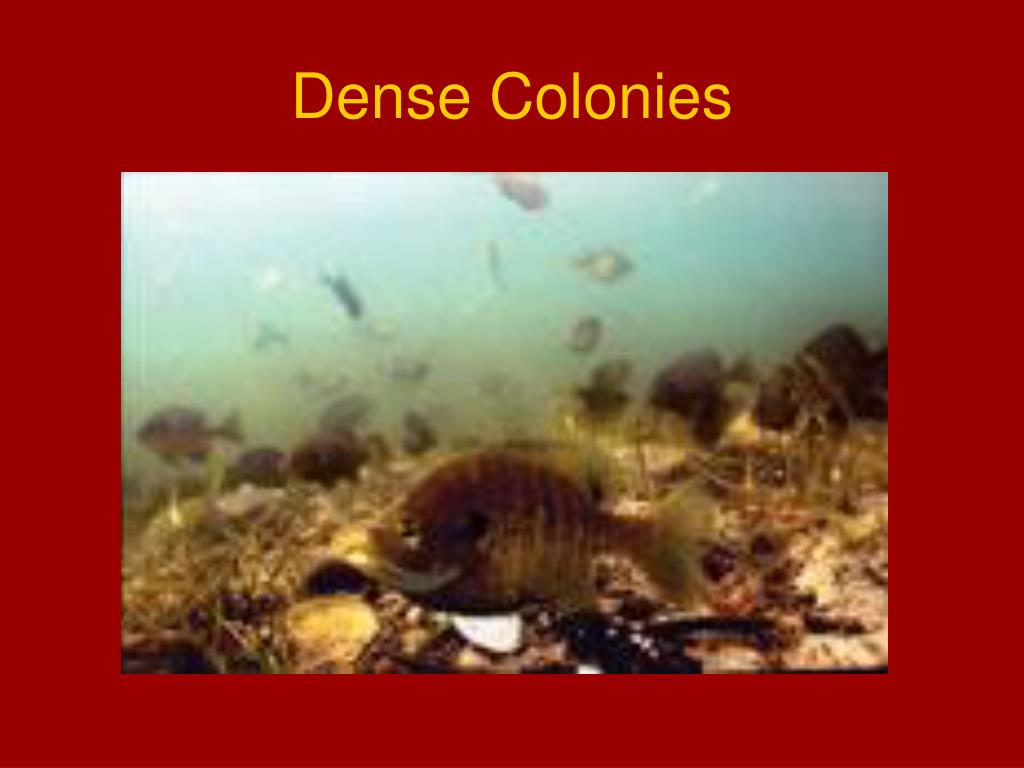This color photograph, presented within a wide maroon border, is titled "Dense Colonies" in yellow text at the top. The image captures an underwater scene with a large brownish fish at its center, surrounded by numerous smaller fish of similar color in the background. The seabed, littered with dirt, debris, and seaweed, adds texture to the setting, while the pale blue water above and below the fish provides a stark contrast. The photo has a grainy quality, likely due to being taken underwater, which gives it a somewhat murky appearance. Despite its blurriness, the large fish is detailed enough to display subtle stripes, a big mouth, prominent eyes, and visible fins. The distant fish, while fuzzier, contribute to the dense, bustling atmosphere suggested by the title.